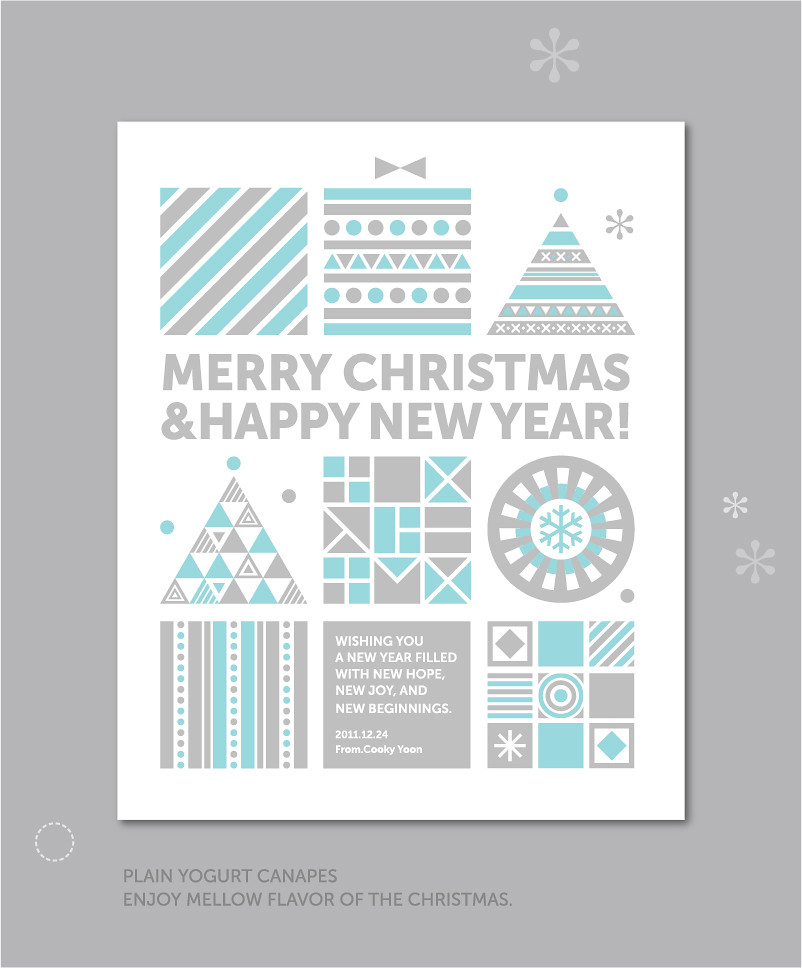The image is a detailed graphic poster styled as a Christmas card, featuring a prominent light gray border with intricate white and gray snowflake designs. The central focus is a greeting in all capital letters, "MERRY CHRISTMAS & HAPPY NEW YEAR!" displayed in a light gray font on a white background. Above this greeting are two squares representing Christmas gifts, a triangle signifying a tree, and a snowflake to the right of the triangle. Beneath the greeting are more geometric shapes: a triangle on the left, a square, and a circle with a snowflake in the center, followed by three additional squares. The card design uses white, gray, and turquoise colors for its geometric elements. At the very bottom of the card, within a gray box, is a heartfelt message in white font: "Wishing you a new year filled with new hope, new joy, and new beginnings," followed by an unclear signature. Additionally, there is an unusual phrase on the border that reads, "plain yogurt canopies, enjoy mellow flavor for the Christmas."